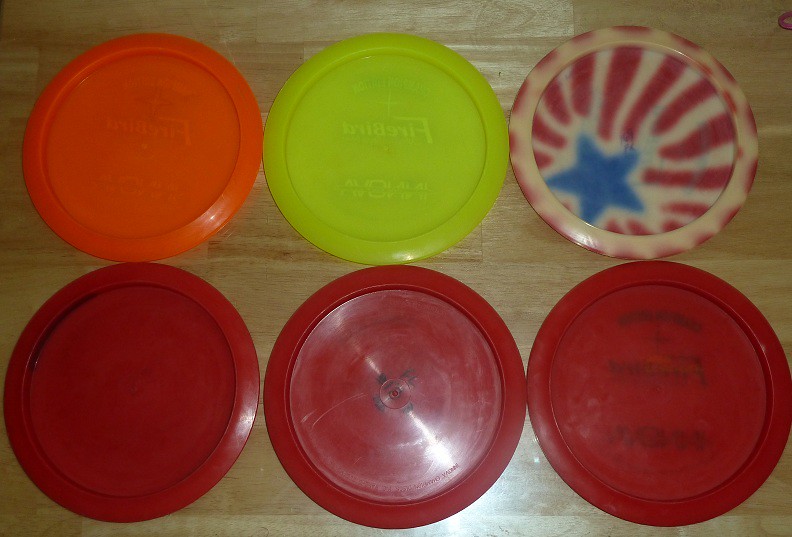The image depicts a collection of six circular plastic Frisbee tops arranged horizontally on a light tan wooden floor. In the top row, from left to right, there is a bright orange Frisbee with reverse lettering that reads "Frisbee," followed by a lime-green Frisbee which also displays the reversed text, and finally, a white Frisbee featuring a decorative design of a hazy blue star with red and white stripes emanating from it. The bottom row consists of three uniformly deep red Frisbee tops, with the one on the far right displaying black reversed lettering that reads "Frisbee." The Frisbee tops are notably scuffed, particularly the lime-green one, which has a prominent scratch on its surface. The light source, a bright white light, illuminates the scene from behind the viewer, casting a reflective glow, especially noticeable in the center of the Frisbees.